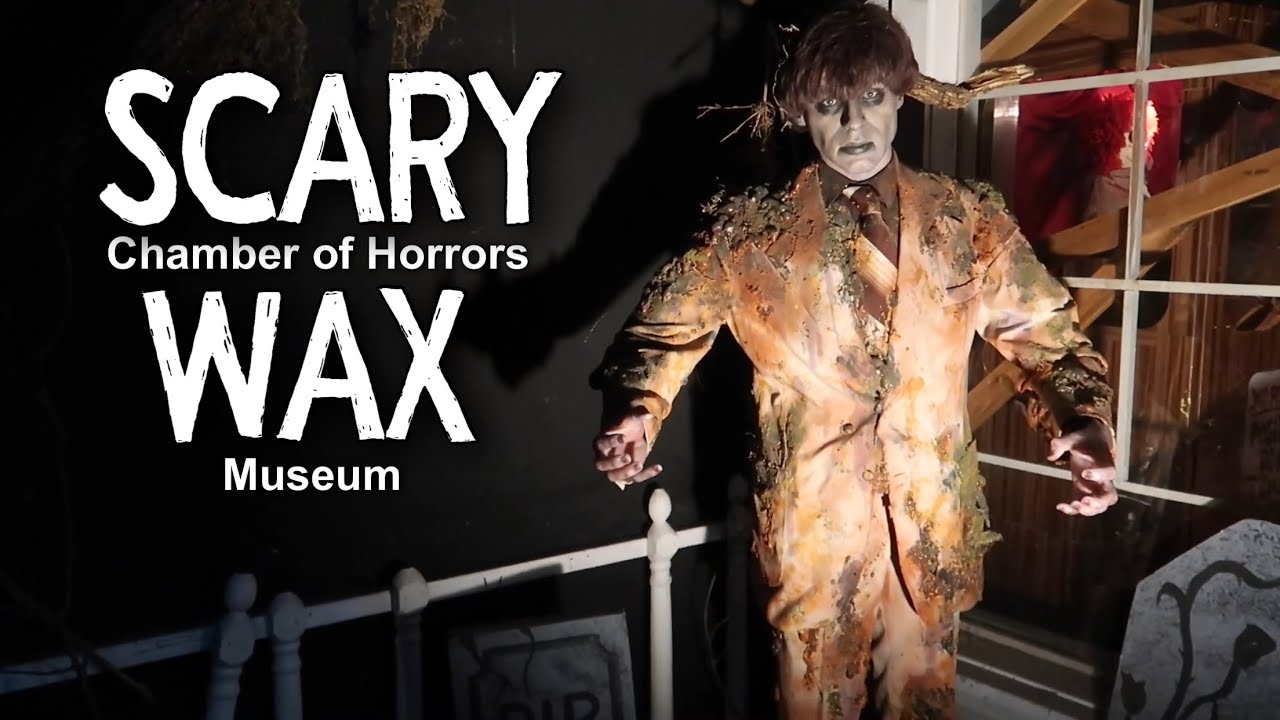The rectangular advertisement for the Scary Chamber of Horrors Wax Museum features a dark, ominous background on the left, with large white lettering that reads, “SCARY CHAMBER OF HORRORS WAX MUSEUM.” The text is styled to resemble a guardrail or fireplace grill, with white and gray colors. In the center, a full-length wax statue of a zombie man dominates the scene. The statue, depicting a man in his 20s to 40s, is dressed in a disheveled, tattered, and soiled tan suit with a dark brown and gold striped tie. His suit appears ripped and chewed, reinforcing his undead appearance. He has reddish auburn hair reminiscent of a Beatles haircut from the 60s, pale ashen skin, and dark circles under his deadpan eyes, which stare hauntingly at the viewer. The wax figure’s left hand grasps the inner framework of a window on the right side of the image, where the glass is missing, revealing red-lit beams of what appears to be a collapsed house. The eerie scene is dimly lit, with the left side of the image shrouded in darkness, contributing to the overall horror theme of the advertisement.